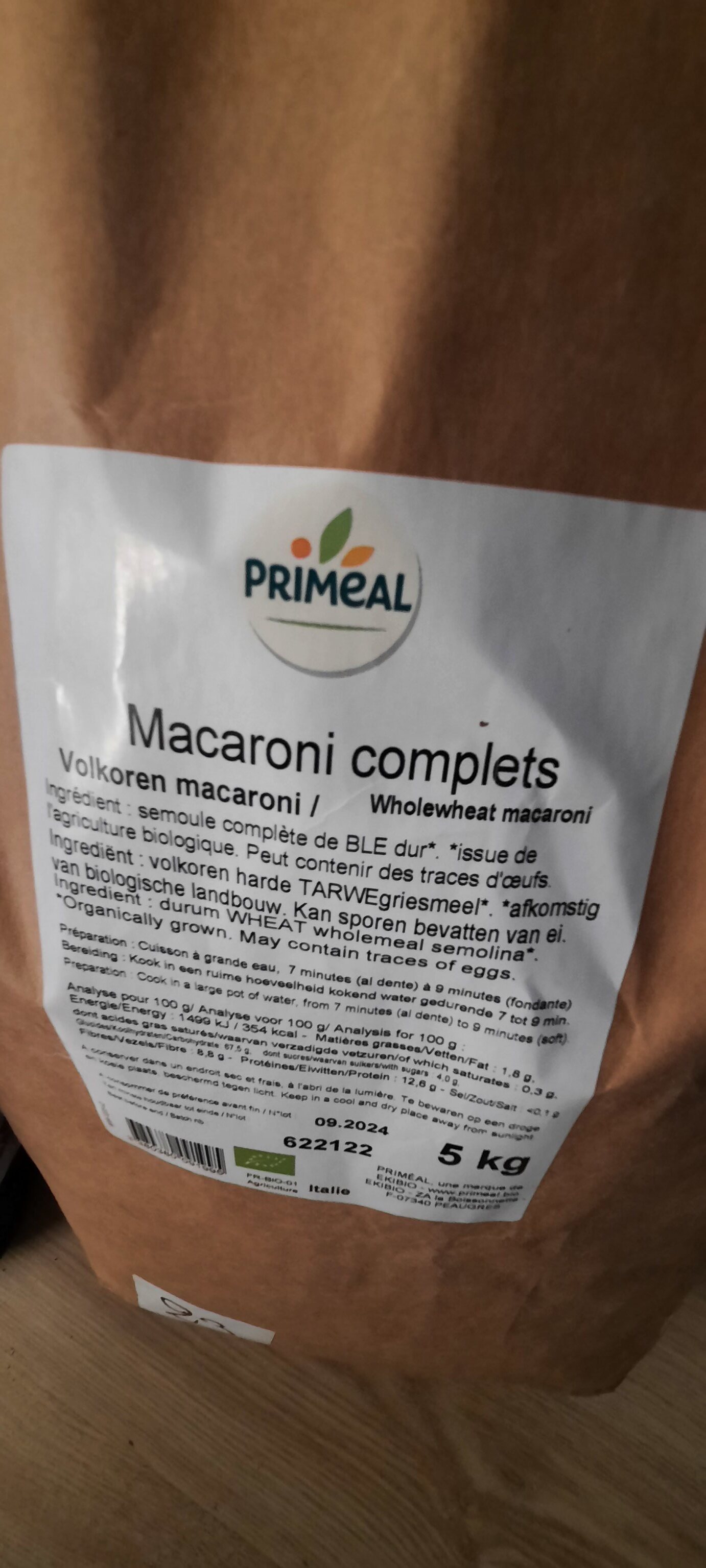The image showcases a brown paper bag package, reminiscent of being positioned on a wooden table. The dominant label on the bag reads "Prime Meal" in blue lettering, accompanied by a decorative motif of intertwined leaves in pink, green, and orange, suggesting a floral appearance. Below this, in black text, multiple references to macaroni are made, including "Macaroni Complex," "Volkorin Macaroni," and "Whole Wheat Macaroni." Additionally, a salient feature is the orange circle positioned on the left side of the label. While the ingredients are present, they are not clearly legible. Noteworthy details also include a green stamp, a barcode on the bottom left, and packaging instructions hinting at recyclability or reusability. Located at the center is the number "622122," and the bottom right of the label specifies the package weight as 5 kg. Furthermore, a white and black label provides cooking instructions, suggesting to cook in a large pot of water for 7-9 minutes, indicating this could be a component of a meal kit or a heat-and-eat meal.